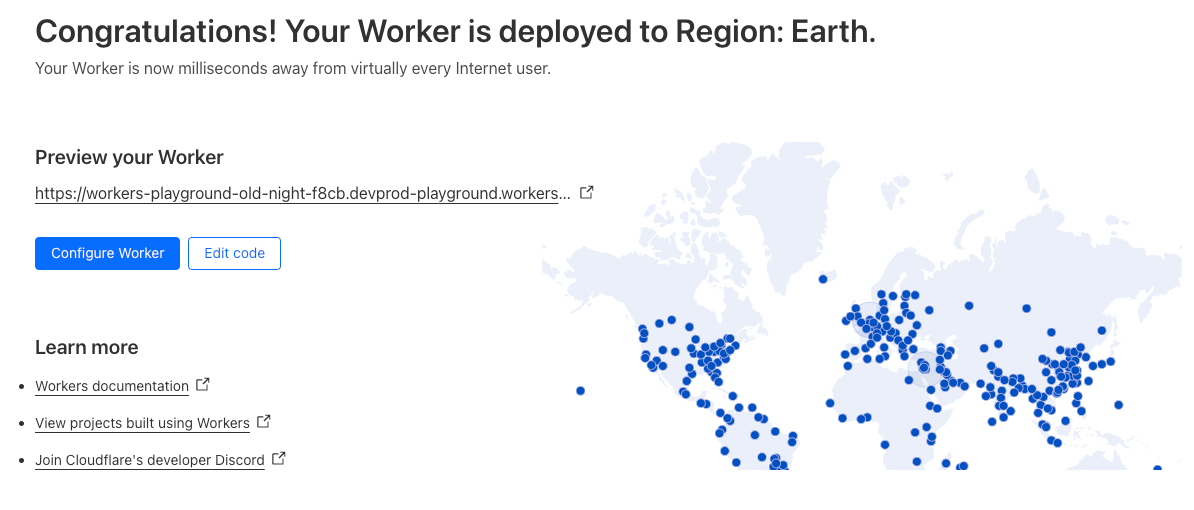Screenshot of a Cloudflare Workers deployment confirmation screen. The prominent text in bold black reads, "Congratulations! Your worker is deployed to region Earth." It further informs that the worker is now milliseconds away from virtually every internet user and includes a link for previewing the worker: [workers-playground-alt-night-fhcp.devprod-playground.workers](https://workers-playground-alt-night-fhcp.devprod-playground.workers). 

There are two key clickable options: a blue button with white text labeled "Configure Worker" and a nearby clickable text in blue on a white background labeled "Edit Code".

Adjacent to these options, on the right side, is a flat, light blue world map densely dotted with many dark blue markers, signifying deployment regions. The markers primarily populate areas outside of Canada, Greenland, Alaska, Iceland, and most of Russia. Concentrations of these markers appear throughout Asia, Europe, the United States, and Northern South America, with a modest presence in Africa.

At the bottom, there are additional resources listed in smaller text: "Learn more about Workers documentation", "View projects built using Workers", and an invitation to "Join Cloudflare Developer Discord".